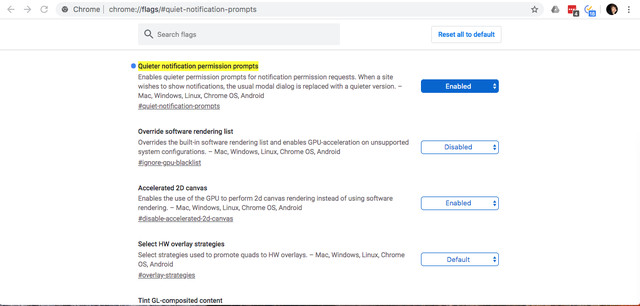The image showcases an interface from the Chrome browser's "Flags" settings page, specifically detailing the "quieter notification permission prompts" setting. 

At the top, the browser's navigation bar features a white background. On the left side, it includes a back button, a forward button, and a refresh button, all appearing disabled in light gray. Next to these, there's an address bar; towards the left of the address bar is a dark gray Chrome logo followed by the word "Chrome" in gray. A lighter gray divider line separates this from the URL, which reads "chrome://flags/#quiet-notification-prompts" with the text "flags" in bold, and the rest in regular font.

Transitioning into the main part of the page, at the top center but slightly towards the left, there's a rectangular search bar with a light gray background. This search bar features a medium gray magnifying glass icon on its left and the words "Search flags" in medium gray text on the right. 

To the right, there is a white rectangular icon with a light gray border containing bold blue lettering that reads "Reset all to default." A gray line runs horizontally across the entire page, serving as a divider.

Below this divider is a blue bullet point accompanied by highlighted black text that reads "Quieter notification permission prompts." A smaller, gray text underneath explains: "Enables quieter permission prompts for notification permission requests. When a site wishes to show notifications, the usual modal dialog is replaced with a quieter version - Mac, Windows, Linux, Chrome OS, Android." 

Finally, towards the right side of this description, there's a dropdown menu with a blue background. In its center, it displays the word "Enabled" in bold white lettering.